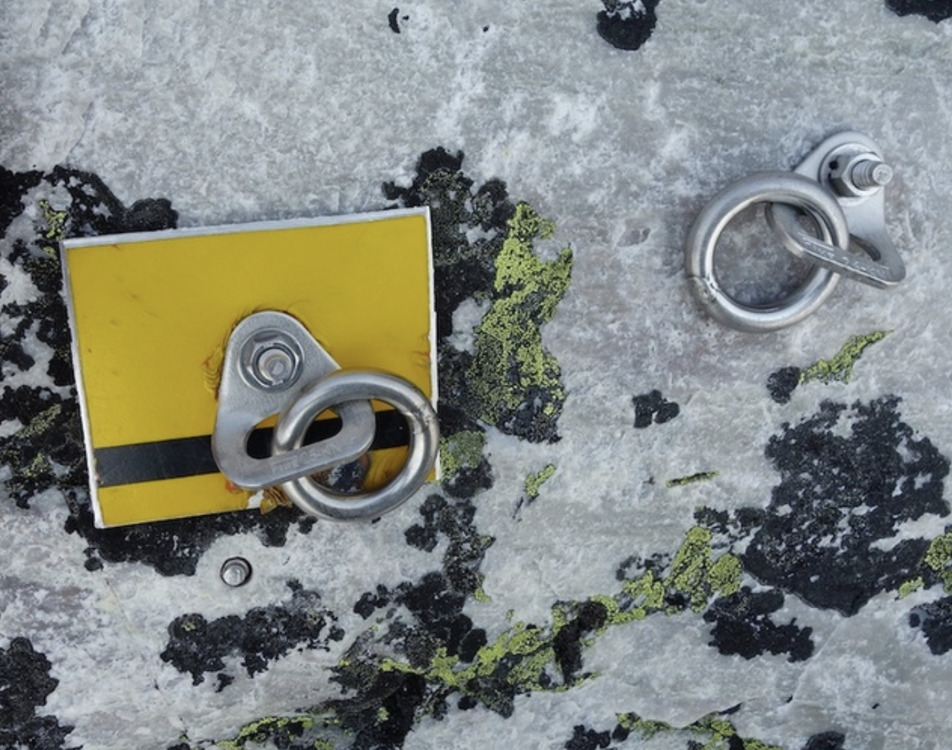This close-up photograph depicts a section of a mottled gray and white stone or cement surface, sparsely populated with bright green and gray lichen, primarily clustered towards the bottom two-thirds of the image. Bolted into this surface are two metal anchor brackets situated side by side. On the left-hand side, there's a distinctive yellow rectangular tab with a gray horizontal stripe near the bottom. At the center of this tab, an L-shaped angle fastener is bolted into the stone, holding a sturdy, welded-shut circular ring. The weld is visible on the right-hand side of the ring. Contrasting this, the right-hand anchor features another bolted L-fastener, similarly equipped with a welded circular ring. Here, the nut end of the bolt is visible rather than the head. These metal brackets and rings, likely used as lifting points for the stone, are indicative of fixtures seen on job sites for moving large rocks or heavy materials.